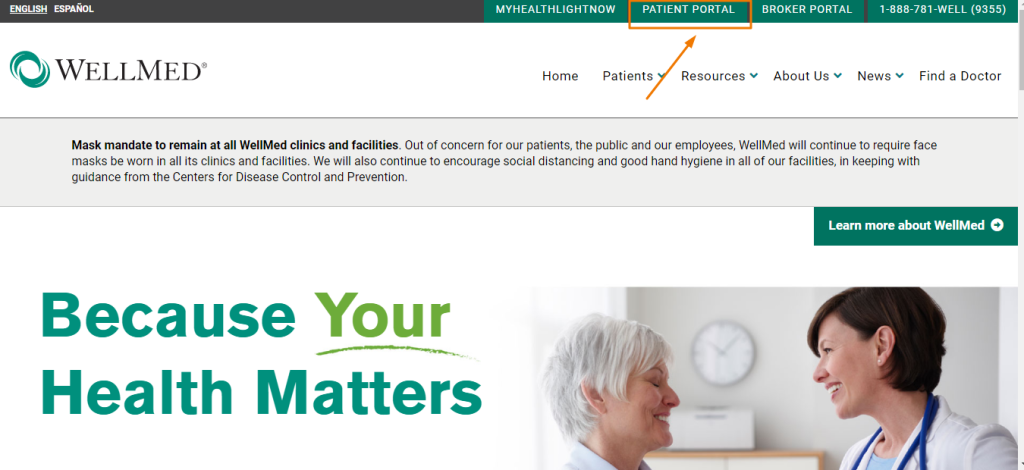This photograph showcases a website interface in great detail. At the very top, there's a sleek, thin rectangular header with a dark black background. On the left side of this header, "English" and "Español" are displayed in white text. Spanning from the center to the right, there are four turquoise rectangles with labels in white font: "My Health Light Now," "Patient Portal," "Broker Portal," and a toll-free number at the far right, 1-800.

Below this, a second header features a vibrant green, 3-D logo designed as a diagonally oriented circle. To the right of this logo, "WellMed" is prominently written in black letters. On the upper right side of this header, there are several drop-down menus titled "Home," "Patients," "Resources," "About Us," "News," and "Find a Doctor."

Dominating the main section of the website, a large, bold green headline reads, "Because Your Health Matters," with the word "your" uniquely underlined in an olive green shade, adding emphasis.

In the bottom right corner of the photo, a compassionate interaction is depicted: a woman doctor, dressed in a white lab coat, is speaking with an older lady who has gray hair. Both women have short hair, engaging in what appears to be a heartfelt discussion, encapsulating the caring essence of the website's message.